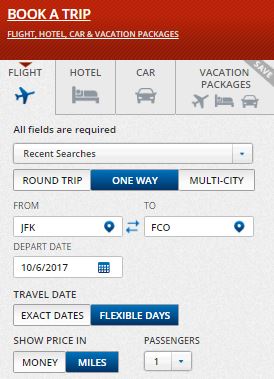This image is a detailed screenshot from a booking application or website, showcasing its user interface. At the top left corner, the phrase "Book a Trip" is clearly displayed in bold white text with an underline, emphasizing the feature. Below this, there are navigation options for different services: "Flight," "Hotel," "Car," and "Vacation Packages," each also underlined in white against a prominent red background, indicating the active selection.

Below the navigation bar, the interface is divided into four main categories, each represented by both text and icons. From left to right, the categories are: 
1. "Flight," marked by a downward pointing red arrow and a blue airplane icon.
2. "Hotel," accompanied by an icon of a bed.
3. "Car," represented by an icon of a car.
4. "Vacation Packages" on the far right, which has a note "Save" in the top right corner and is illustrated with icons of a plane, a bed, and a car, indicating a combination of services.

Centrally located on the page is a form prompting users to fill in their trip details. It clearly states that "All fields are required." The example fields shown in the image are for a flight from "JFK" (John F. Kennedy International Airport) to "FCO" (Leonardo da Vinci–Fiumicino Airport). The departure date is specified in a box as "10-6-2017," illustrating how users should input their travel information.